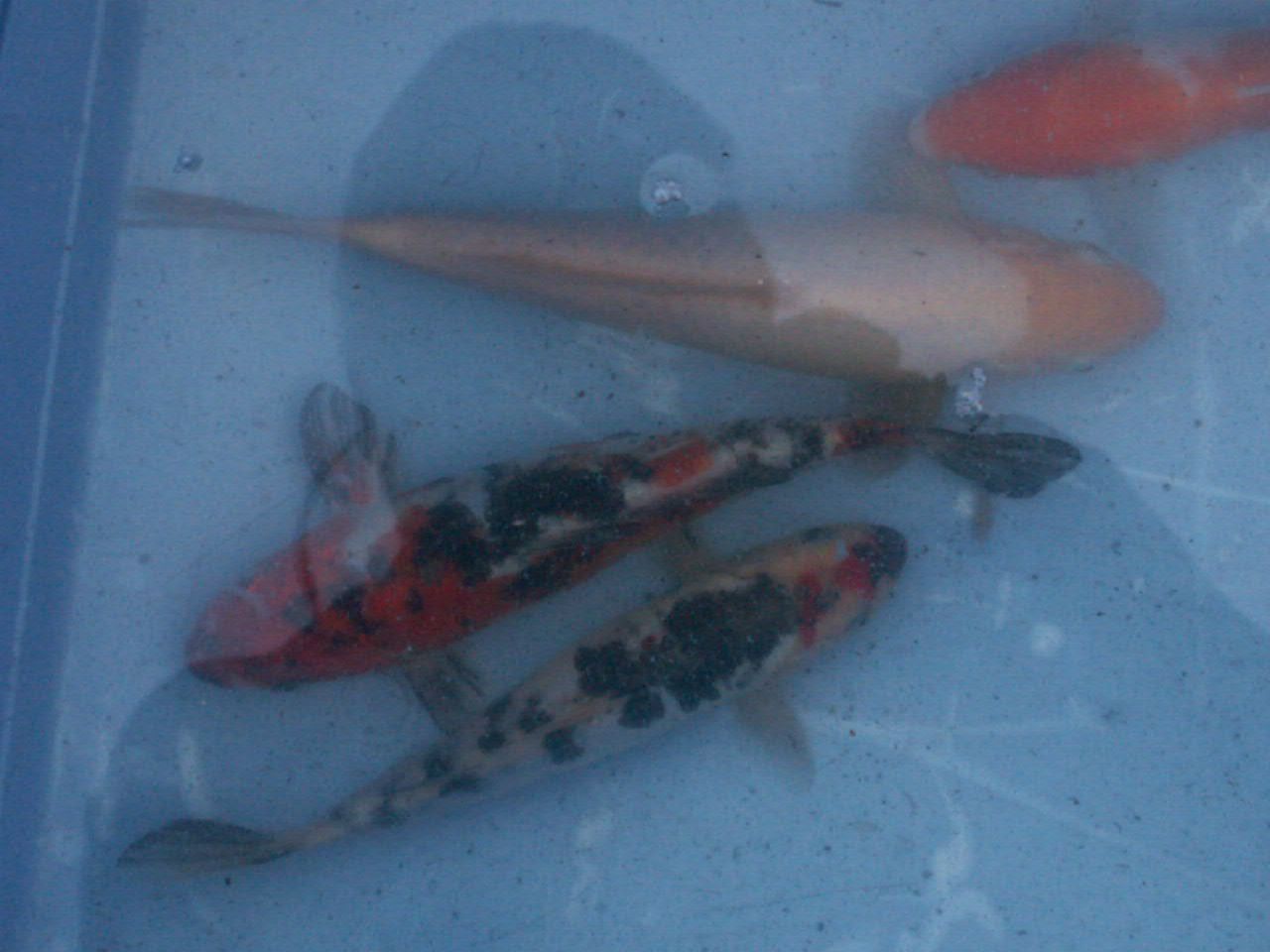This is an amateur, slightly grainy photograph taken from a bird's eye view of a shallow, artificial pond with a plain blue bottom and some specks of sediment. The photograph captures a small pool of water that appears to be clean. The shadow silhouette of the photographer is visible in the middle of the image, slanted toward the bottom right. There are four fish in total, each uniquely marked. One fish at the top right, partially cut off, is colored bright orange with white piebald spots along its side. Another fish positioned about a third from the top, facing to the right, has a gradient coloring with a medium brown tail, lighter brown body, and a golden head. In the lower part of the image, around 8 o'clock, there is a fish with an orange head, white tail, and black spots. Moving further down, another fish swims in the opposite direction to this one, showcasing a predominantly white body adorned with orange and black spots.